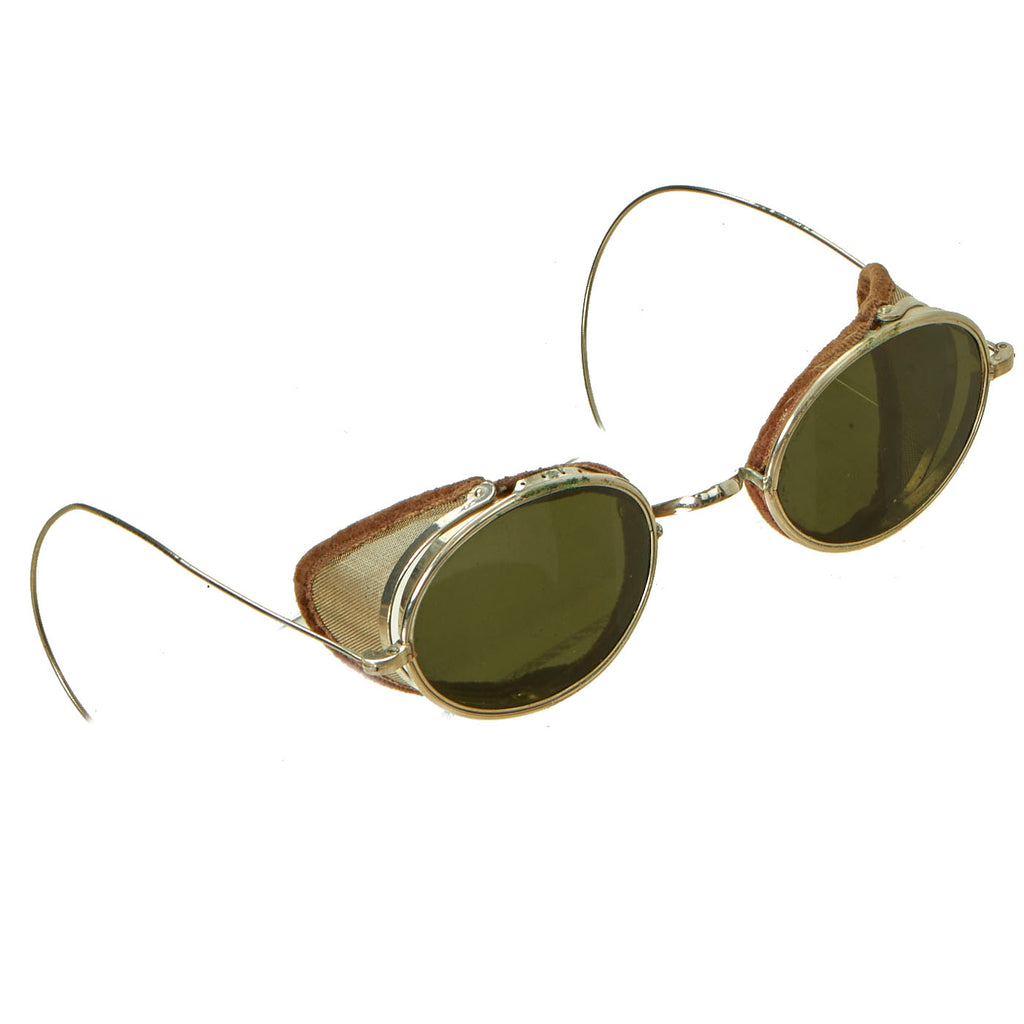This high-resolution image depicts a pair of old-fashioned aviator sunglasses or goggles, set against a plain white background with no visible borders, providing a clean, professional appearance. The sunglasses have round, slightly oval lenses with a grayish-green tint, suggesting their use as protective eyewear. These lenses are bordered by a thick frame that resembles meshed metal, with light brown grid-like enclosures extending to the sides to fully cover the eyes and block peripheral light. 

The frames are connected by a single silver metal bridge at the nose, and the thin, polished silver metal ear hooks extend diagonally towards the upper left of the image, while the lenses face towards the lower right. For added comfort, the goggles feature a darker brown, fuzzy cushioning on the inside. Despite their age, the sunglasses are preserved relatively well, evoking the old-world charm of vintage aviation gear. The image, absent of any writing or additional elements, focuses entirely on these meticulously detailed, reflective artifacts.